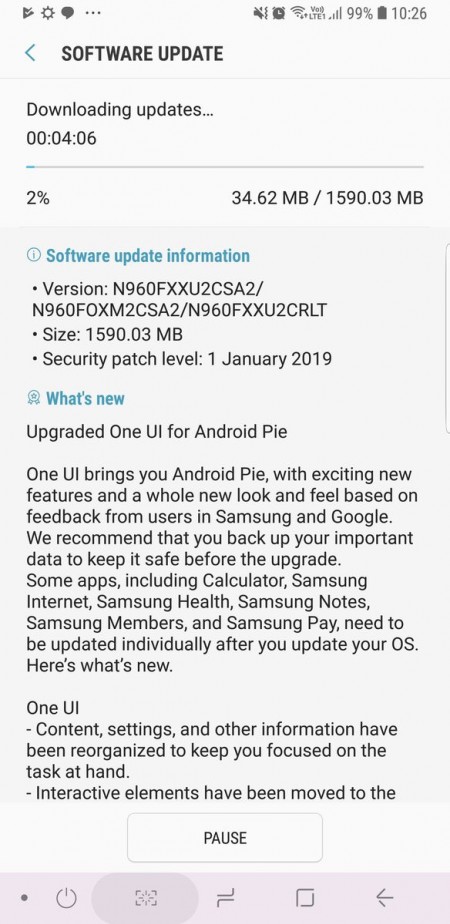This screenshot captures a cell phone's software update notification. The background is a light grayish-blue color. At the top left corner are various phone icons, including a gear icon, a sideways triangle with a checkmark, and a text message bubble. Three vertical dots indicate more options. On the top right, the notification bar shows a sound speaker icon with a line through it, indicating the phone is on silent, along with icons for an alarm, internet, LTE connectivity, and the battery level at 99%. The time displayed is 10:26.

Below the notification bar, bold black letters spell out "Software Update," with a blue arrow pointing left on its left side. The update status below it reads "Downloading updates" with an estimated time of four minutes and six seconds remaining. A progress bar below indicates the download is at 2%, specifically 34.62 megabytes out of the total 1590.03 megabytes.

Further details in blue text read "Software Update Information," followed by bullet points listing the version, size, and security patch level of the update. Below, a blue section titled "What's New" details upgrades, including "Upgraded One UI for Android Pie." More bullet points discuss collaboration between Samsung and Google and additional updates for One UI.

At the bottom of the screen, there’s a pause button and a series of icons, including an arrow and what appears to be a timer, among other unclear symbols.